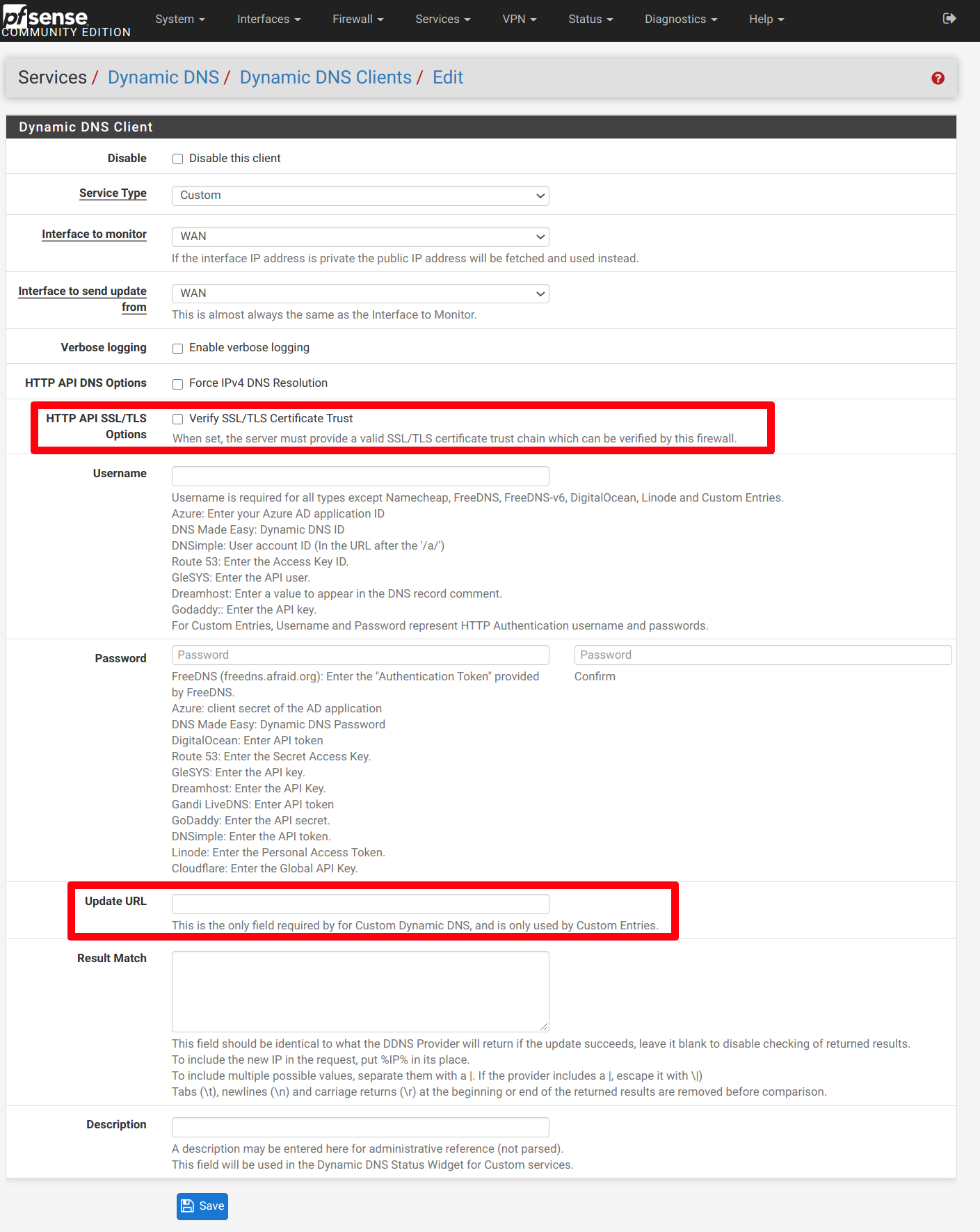**Instructional Screenshot: Configuring Dynamic DNS in PFSense**

This screenshot captures the dynamic DNS configuration page within the PFSense Community Edition web interface. At the top, the interface features a distinctive black banner displaying the "PFSense Community Edition" text alongside the PFSense logo. The banner also includes multiple categories with accompanying drop-down menus for effortless navigation.

Below the top banner, a gray navigation bar displays the breadcrumb trail: "Services > Dynamic DNS > Dynamic DNS Clients > Edit," indicating that the user is currently on the Edit screen.

Central to the screenshot is a white content area titled "Dynamic DNS Client," encapsulated by a black header. This section comprises various configuration options, including drop-down menus and checkboxes. Among these, the "HTTP API SSL/TLS Options" category is conspicuously highlighted with a red border, signifying its importance. Furthermore, towards the bottom of this section, the "Update URL" field is similarly emphasized with a red box, directing attention to key elements that require user action.

To facilitate the user, annotations using red boxes have been added to highlight essential options that need to be selected or configured. This visual aid ensures that users can easily follow the necessary steps.

At the bottom left corner of the page, a blue "Save" button is available for users to apply their changes and finalize the configuration.